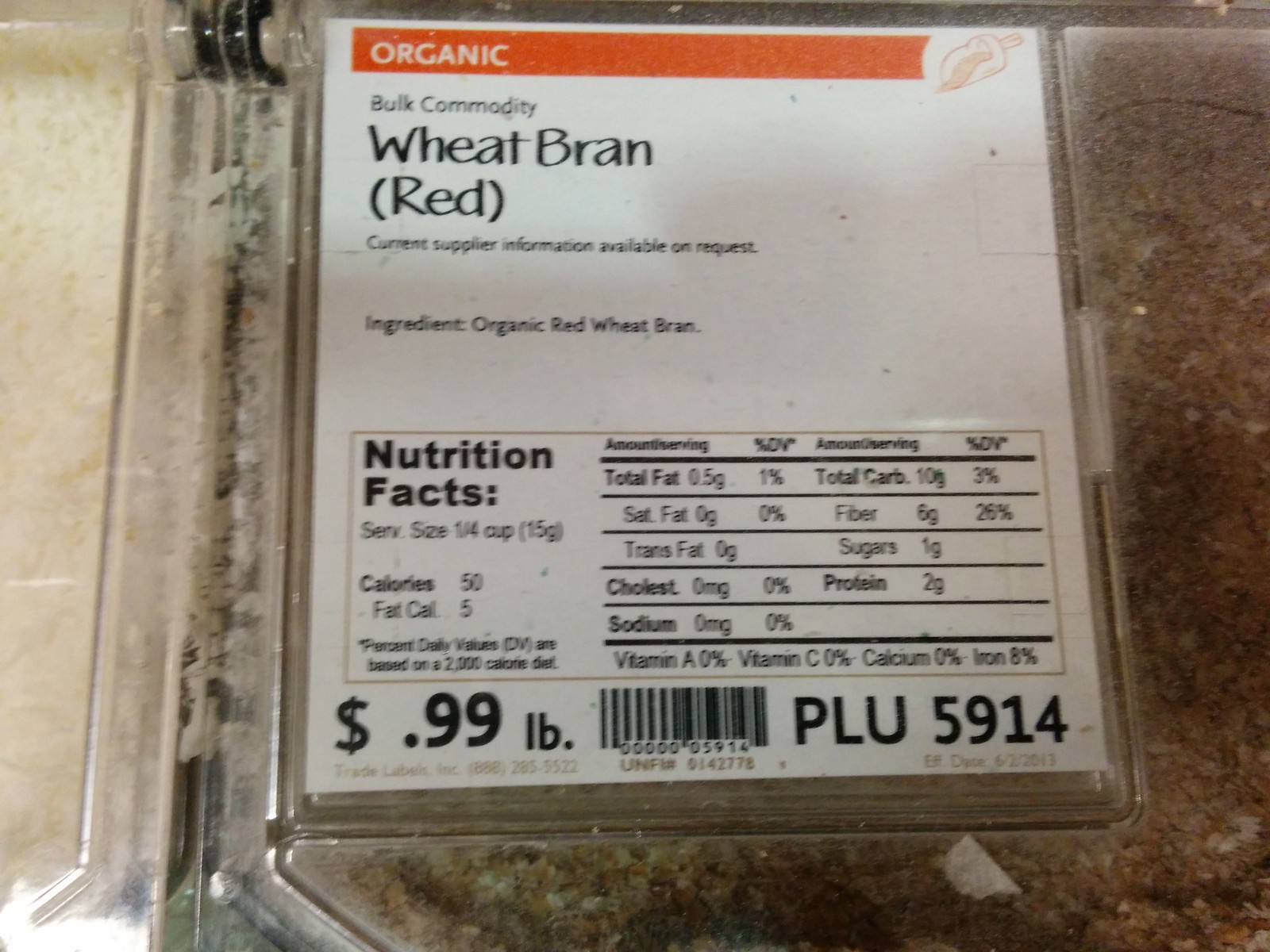The image features a nutrition label affixed to a bulk commodity bin. Dominating the top of the label is a prominent orange line running horizontally from the left to the right, emblazoned with the word "ORGANIC" in uppercase letters. Below this banner, the label identifies the product as "Bulk Commodity Wheat Bran (Red)." In smaller print, it notes that current supplier information is available upon request. The ingredient is specified as "Organic Red Wheat Bran."

Detailed nutritional information is provided, with a serving size listed as a quarter of a cup (15 grams), containing 50 calories, of which 5 calories are from fat. The price is indicated as 99 cents per pound. Additionally, the label includes an item code for inventory purposes: POU5914. The design and textual details suggest a clear, organized label, aimed at providing essential information to the consumer efficiently.